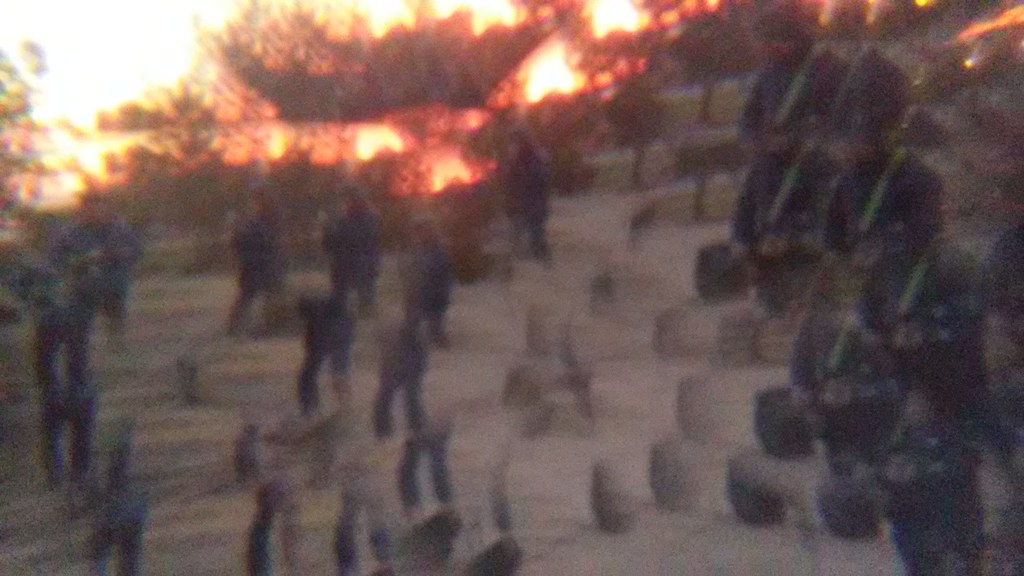The image is a blurry and low-quality photograph that evokes a kaleidoscope effect, causing the figures within to appear duplicated and scattered across the scene. Central to the composition are three main individuals: a man holding a newspaper, a young woman in a blue jumpsuit, and a young man in a similar blue jumpsuit, distinguished by a green strap or belt across his shoulder. These people are positioned on the left side of the image, seemingly indifferent to their surroundings as they wave. Behind them, a striking backdrop features a tree line engulfed in flames, with vivid red and yellow hues lighting up the sky. The lower part of the image reveals multiple legs, contributing to the chaotic overlay. To the right, indistinct blocky objects in black and grey add to the confusion. Their faces are nearly indistinguishable due to the image's poor resolution. Overall, the scene is surreal, combining elements of repetition, vibrant fire colors, and a sense of disarray.